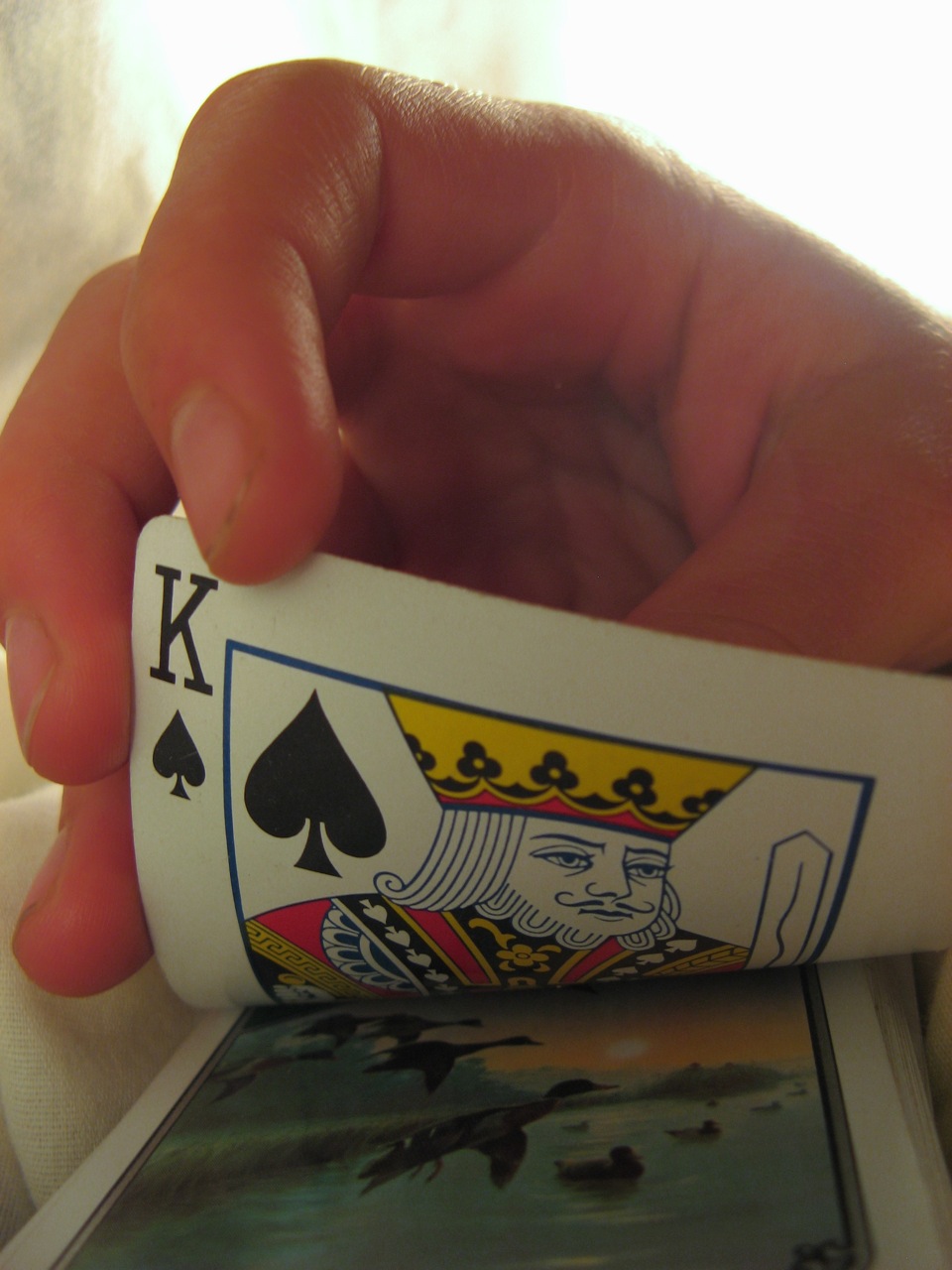In an indoor setting, a photograph captures a close-up view of a person's hand resting on a surface, holding a partially revealed King of Spades playing card. The card is held upright, prominently displaying the 'K' and the iconic spade symbols in black. The intricate design of the king character is visible in the middle of the card. 

Beneath the King of Spades, another card is partially seen, showcasing a tranquil scene of a lake surrounded by bushes and grass, with a few birds flying and floating on the water's surface. The background is brightly lit, enhancing the visibility of a white area in the upper left corner. The entire image is framed in a rectangular shape, bringing a focused yet detailed perspective to the diverse elements within the scene.